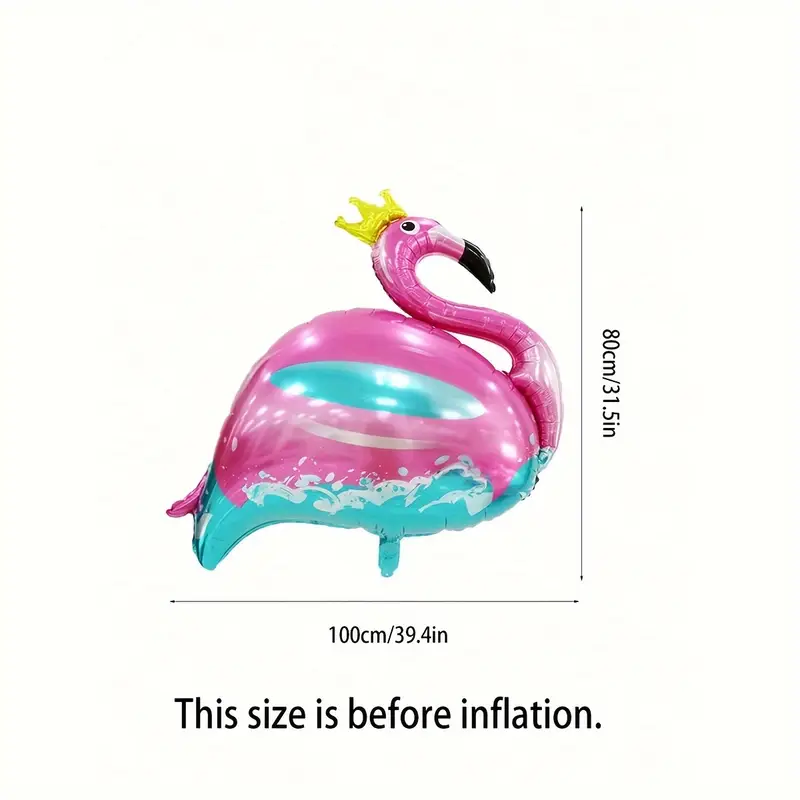The image features a detailed measurement chart of an inflated mylar flamingo balloon adorned with a gold crown. The pink flamingo, facing to the right, has teal-blue coloration at the bottom of its body, resembling splashing waves. The balloon's black beak and eye stand out against its vibrant colors. On the right side of the image, a vertical measurement indicates the height of the flamingo as 80 centimeters (31.5 inches). Along the bottom, a horizontal line marks the width as 100 centimeters (39.4 inches). Below these measurements, a note in black text reads, "This size is before inflation." The entire image is set against a plain white background.